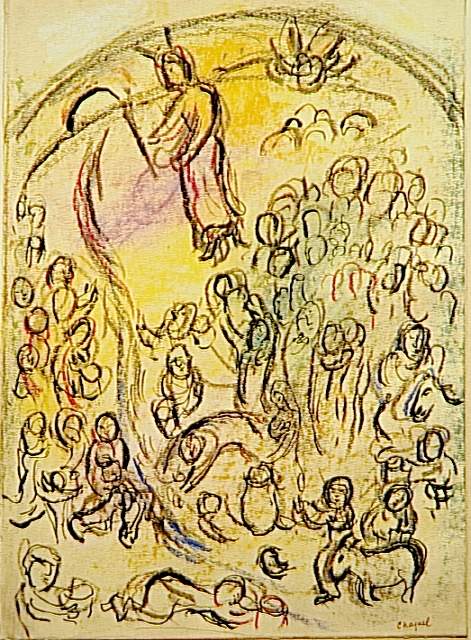This photograph captures a colorful crayon sketch on a white or light taupe background. Dominating the image is a large, arching rainbow that spans from left to right in a semi-circle across the top. Just below and to the left of this rainbow, there appears to be a figure holding something, possibly with antlers or antennae on their head. A meandering path leads towards a sun or a bridge opening on the left side of the sketch. Scattered throughout the drawing are numerous simplistic representations of people, depicted with circles and lines, and a signature can be seen at the bottom right corner, although it’s illegible. Notably present are a few sketched animals, including what looks like a goat and some baby animals, located towards the bottom right. The palette consists of vibrant hues—yellow, blue, red, orange, pink, black, and gray. Despite the whimsical and playful nature, hinting that it might have been created by a child, the drawing occupies the entire space, making it a lively and engaging piece of art.